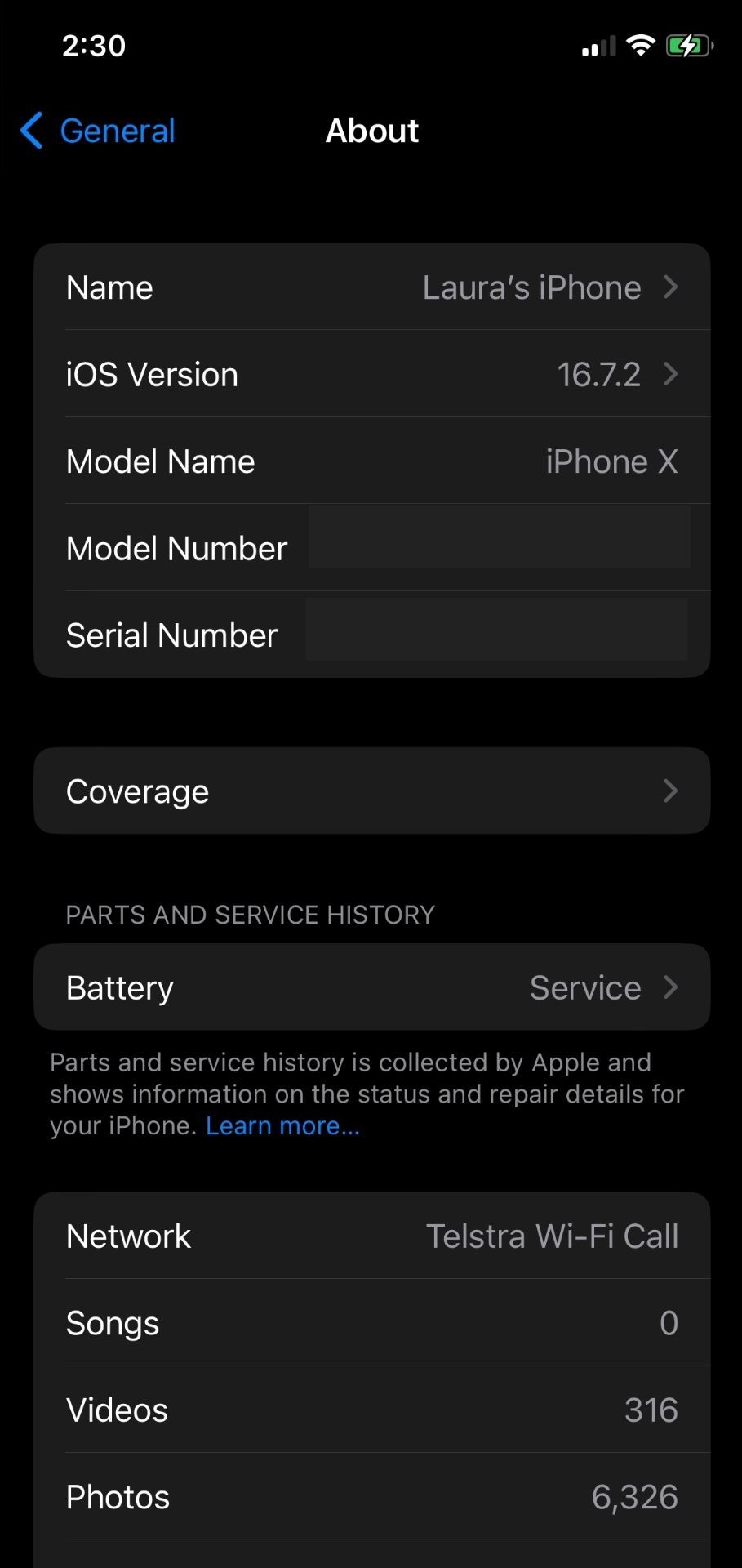This is a detailed screenshot from an iPhone's "About" section under General Settings, displayed in Dark Mode. At the top, the iPhone is named "Laura's iPhone," with an arrow on the right side indicating an option to change the name. The iOS version is 16.7.2, accompanied by an arrow suggesting additional information is available. The iPhone model is identified as an iPhone X. Both the model number and serial number are redacted.

The next section displays "Coverage," followed by "Parts and Service History." Below this, under "Battery," it indicates "Service," with an arrow for more details. A brief note under "Parts and Service History" states that this information is collected by Apple and outlines the status and repair details for the device, including a "Learn More" button.

Further down, four additional sections are listed:
- Network, showing "Telstra Wi-Fi Call."
- Songs, with a count of zero.
- Videos, numbering 316.
- Photos, totaling 6,326.

The interface is in Dark Mode, featuring a predominantly dark gray background with lighter gray text. Main headings such as "Name" are in white, while specific details like "Laura's iPhone" appear in light gray. There is also a blue button to navigate back to the General menu.